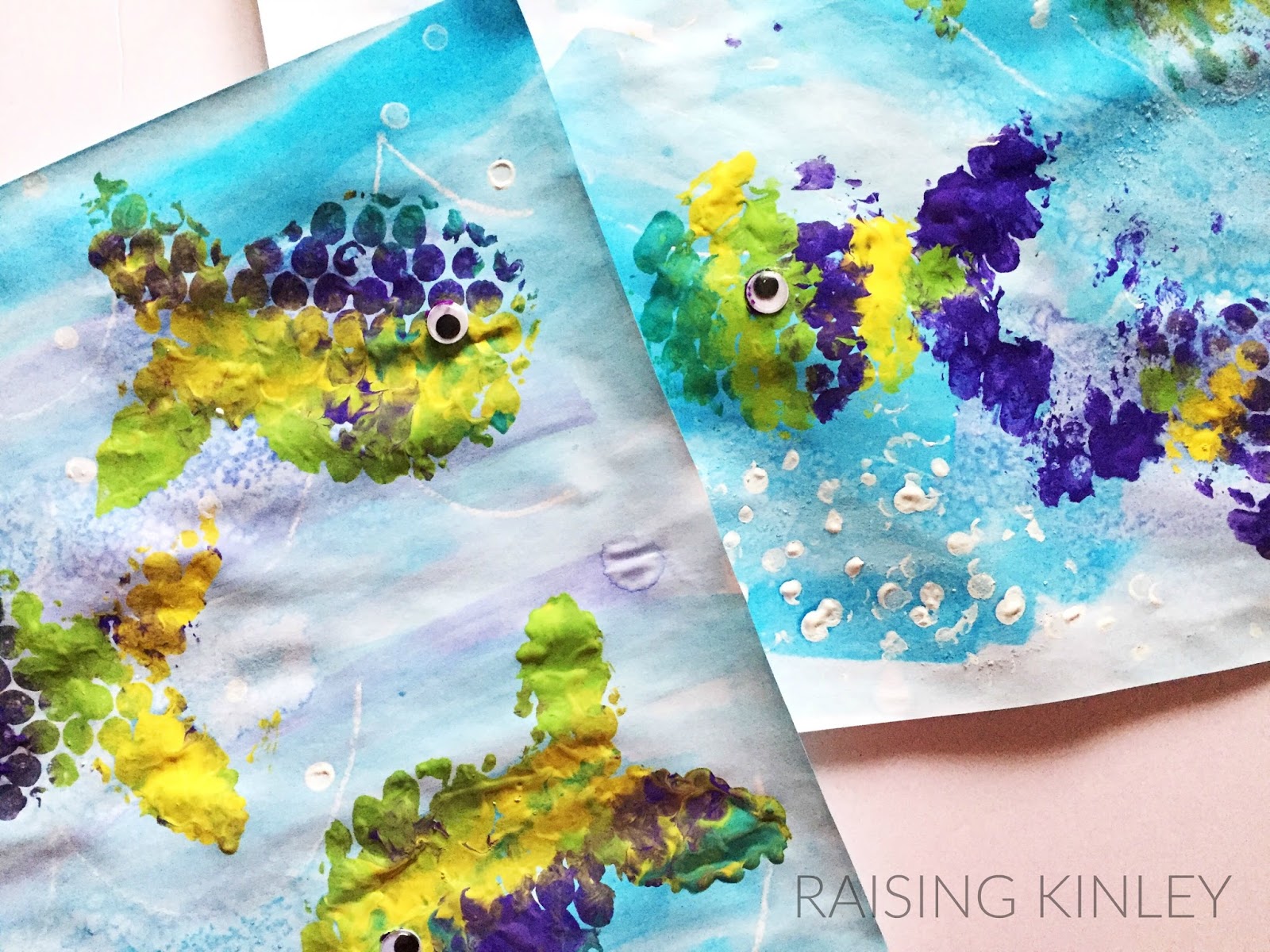The image showcases a child’s art project, likely featured on a family blog named "Raising Kinley," as noted by the watermark on the right-hand side. The artwork consists of two overlapping sheets of paper, placed on a pale pink surface, each adorned with vibrant, textured watercolor paintings depicting a sea scene. The water is rendered in various shades of blue, turquoise, and purple, creating a lush aquatic backdrop. The focal points are the tropical fish, painted in hues of purple, teal, yellow, and green, with distinctive googly eyes and drawn accents to suggest movement. The fish are split between the two sheets: the left sheet displays three of them, and the right sheet shows two. The paintings combine different household materials, including potential elements like salt for added texture, making them an engaging example of a child-friendly craft activity.